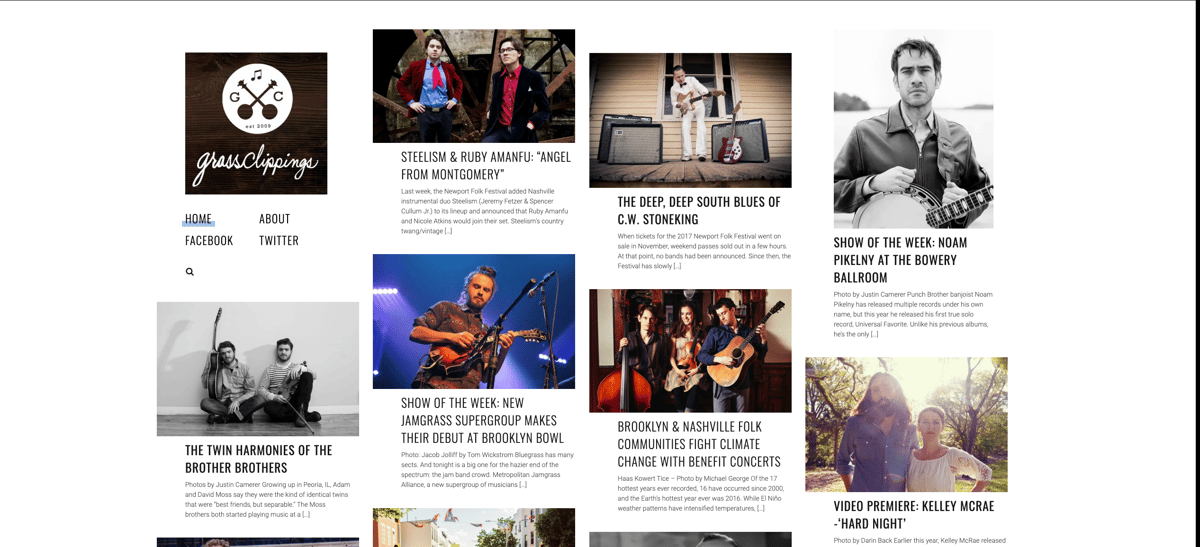The Grass Clippings website showcases offbeat, non-mainstream bands with a focus on bluegrass music. The home page is designed with numerous small rectangular sections, each featuring images of various singers and bands, accompanied by brief descriptions underneath. In the top left corner, there's a distinct black square with the website's name, "Grass Clippings," inscribed in white cursive at the bottom. Directly above this square is a circular logo depicting two crisscrossed banjos flanked by the letters "G" and "C," with a musical note positioned above them.

One highlighted feature on the site is an article titled "The Deep Deep South Blues of C.W. Stone King," which includes a striking image of C.W. Stone King himself, dressed in a white suit and standing next to some amplifiers. Each section of the website offers similar insights and visuals, providing a thorough introduction to various unique and lesser-known musical groups.